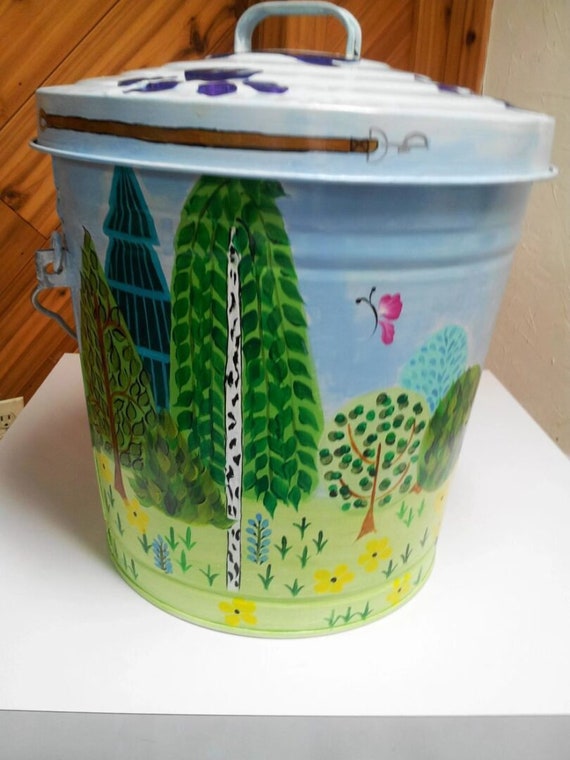The image captures a folk art-styled, small garbage pail, reminiscent of old-fashioned bins from the 70s to 90s. Standing about a foot and a half tall, the pail has a steel body with a handle for carrying, and a removable lid with its own handle. It is placed on a white platform, showcasing its intricate hand-painted design. The scene on the pail features a vibrant and whimsical outdoor motif with a butterfly or dragonfly flying through a blue sky. Surrounding the insect are stylized trees, some painted in blue, green, and light green hues, resembling Christmas trees. Among them grows colorful flora, including yellow flowers and a pink orchid, all set against a backdrop of lush grass and small blooms. The top of the lid is also adorned with flowers, adding to the overall charm and aesthetic appeal of this unique piece.